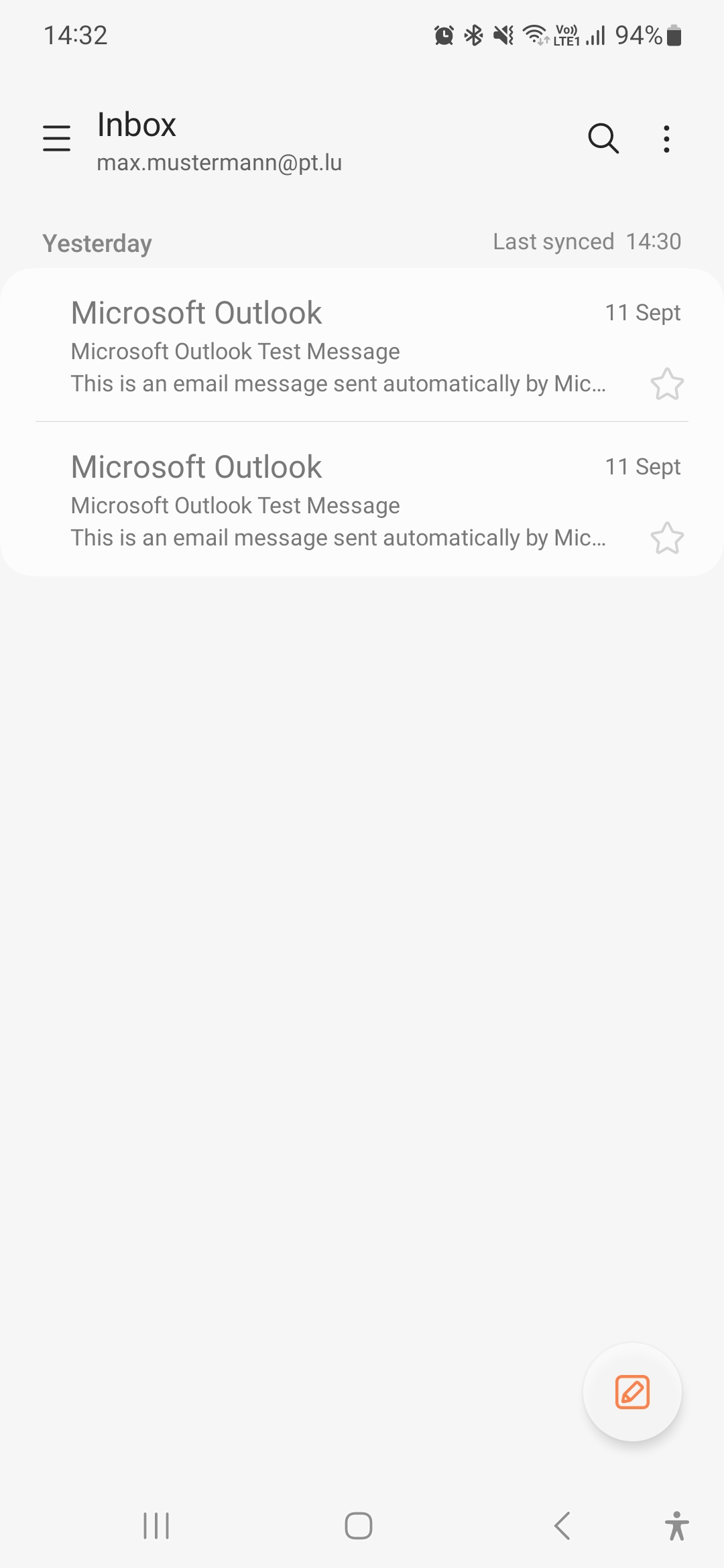The image depicts a smartphone screen displaying an email application, specifically Microsoft Outlook. The current time is 14:32, and several status indicators are visible: there is an alarm icon, a Bluetooth icon, no visible Wi-Fi signal bars, and a battery icon showing 94% charge. The screen is primarily black, gray, white, off-white, and orange in color.

The main content of the display is the inbox, which is under the email address "max.muster@pt.lu". The screen indicates that the inbox was last synced at 14:30 yesterday. The most recent visible email is a test message from Microsoft Outlook, sent automatically on the 11th of September. The message is repeated and cuts off slightly, showing only "MIC..."

At the bottom of the screen, there is an orange circle with a pencil icon inside, which serves as the compose button for creating a new email. Below this button, the phone's navigation bar includes three horizontal lines (possibly a menu or options button), a circle (likely the home button), a back button, and another icon resembling a person in gray, whose function is unclear.

The overall design emphasizes white space, as the inbox contains few items, prominently featuring the test email from Microsoft Outlook and enhancing the minimalist aesthetic of the application.